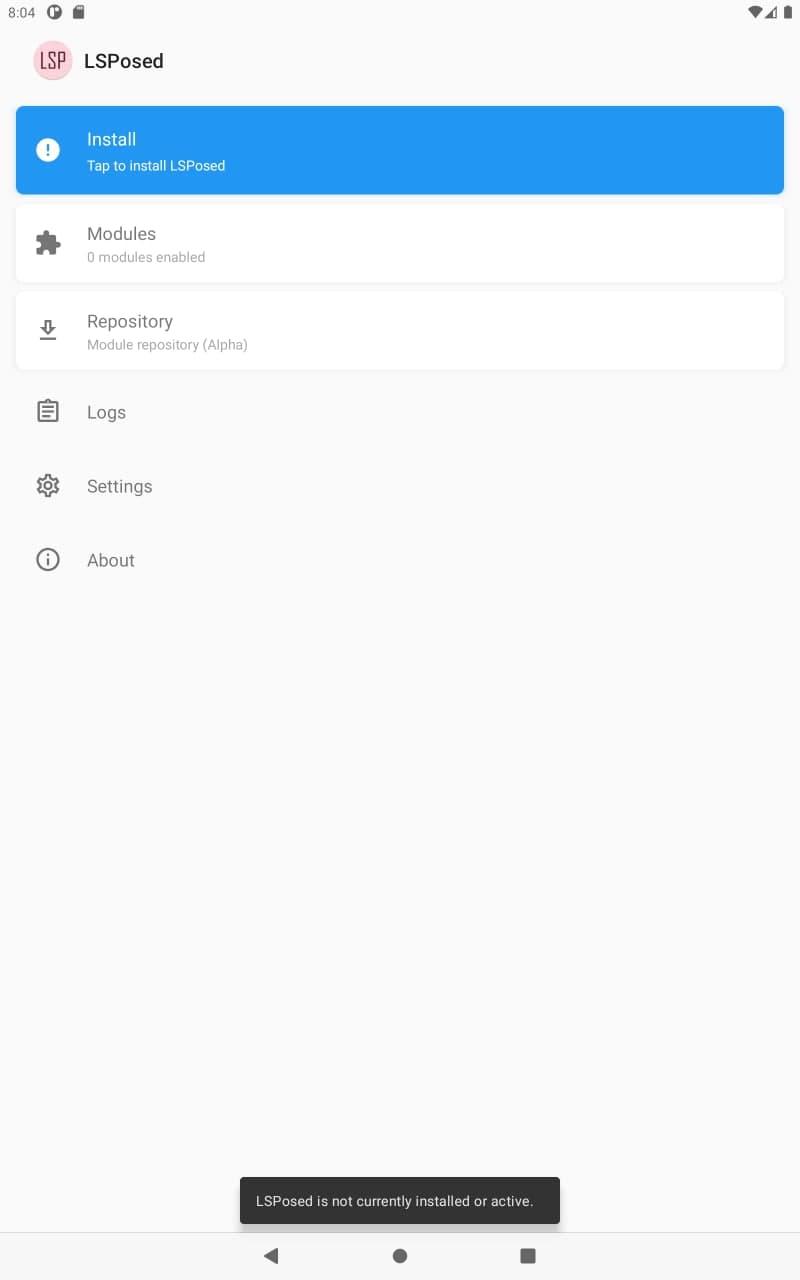A detailed screenshot of a mobile application interface is displayed, showing the user configuring the app called "LSP." The device's status bar at the top indicates the time is 8:04 with two notification icons — one resembling a circular design with shapes inside, and the other a document symbol. On the right side of the status bar, the Wi-Fi, LTE signal, and battery icons are visible without a percentage indicator.

Below the status bar, the app's header displays the name "LSP" against a pink background, accompanied by an instruction to "Install." A blue-highlighted "Install" button with an exclamation point next to it is prominently featured. The interface proceeds to show sections labeled "Modules" with the status "Zero Modules Enabled," and "Repository" with "(Alpha)" in parentheses.

Three additional options are listed under the Repository section: "Logs," "Settings," and "About." The overall color scheme of the app is predominantly white with subtle light gray elements, except for the blue install button. At the bottom of the screenshot, a gray button with a message indicates that "LSP is not currently installed or active."